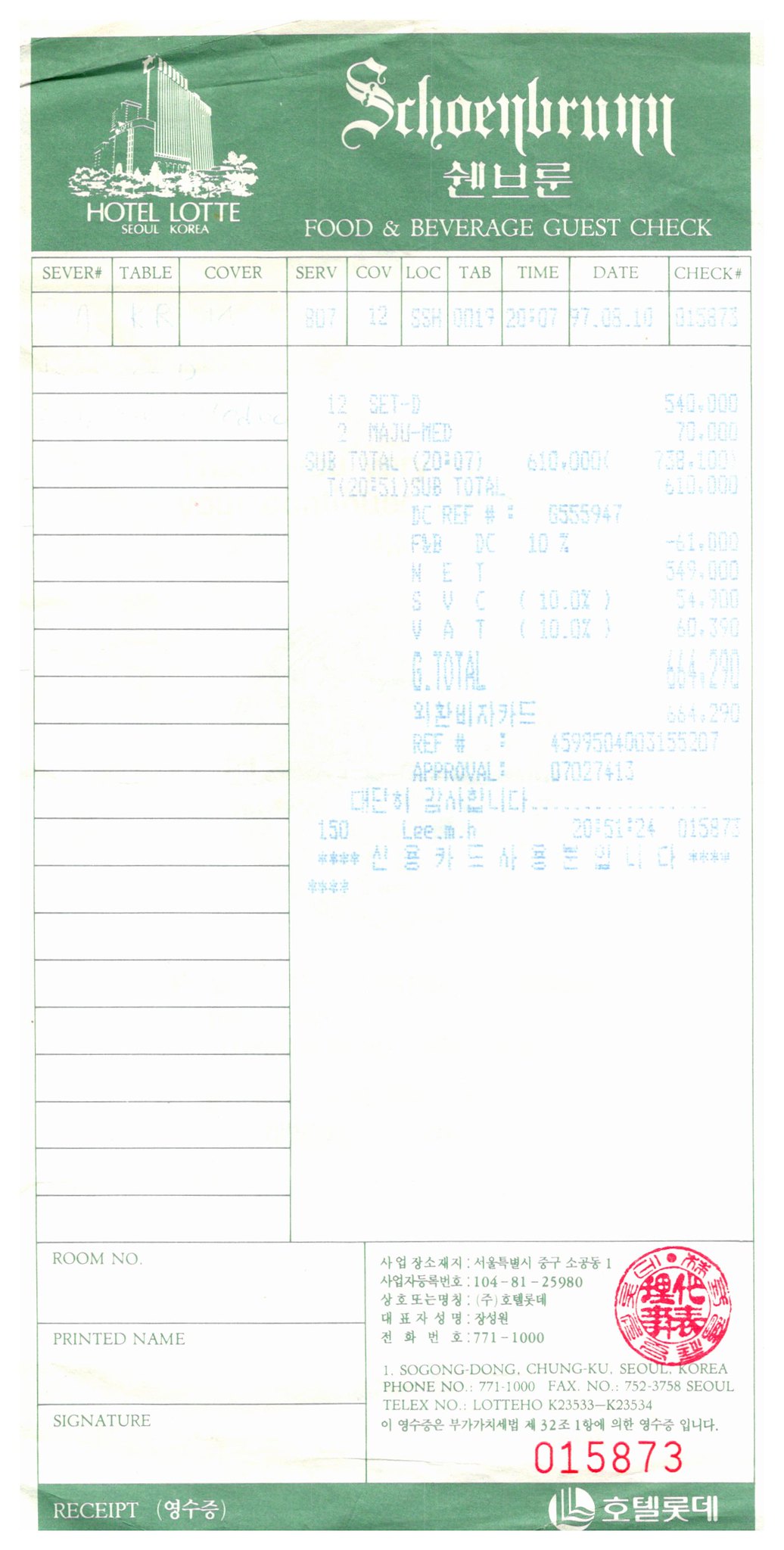The image depicts an old-fashioned hotel receipt from Hotel Lotte in Seoul, Korea, with multiple lines of Korean text. In the top left-hand corner, the hotel name "HOTEL LOTTE" is prominently displayed, followed by "Seoul, Korea." Below this, it states "Food and Beverage Guest Check," indicating it is a bill for food and drink. The bottom right-hand corner of the receipt includes contact information, such as a phone number (771-1000) and a fax number (752-3758), both written in Korean characters. Various text boxes label sections for room number, printed name, and signature. Additional service details like server number, table, cover, serve, COB, LOC, tab, time, date, and check number are present. The total amount of the bill is 664 won, and at the very bottom left, the receipt number is marked within a green-bordered rectangle.